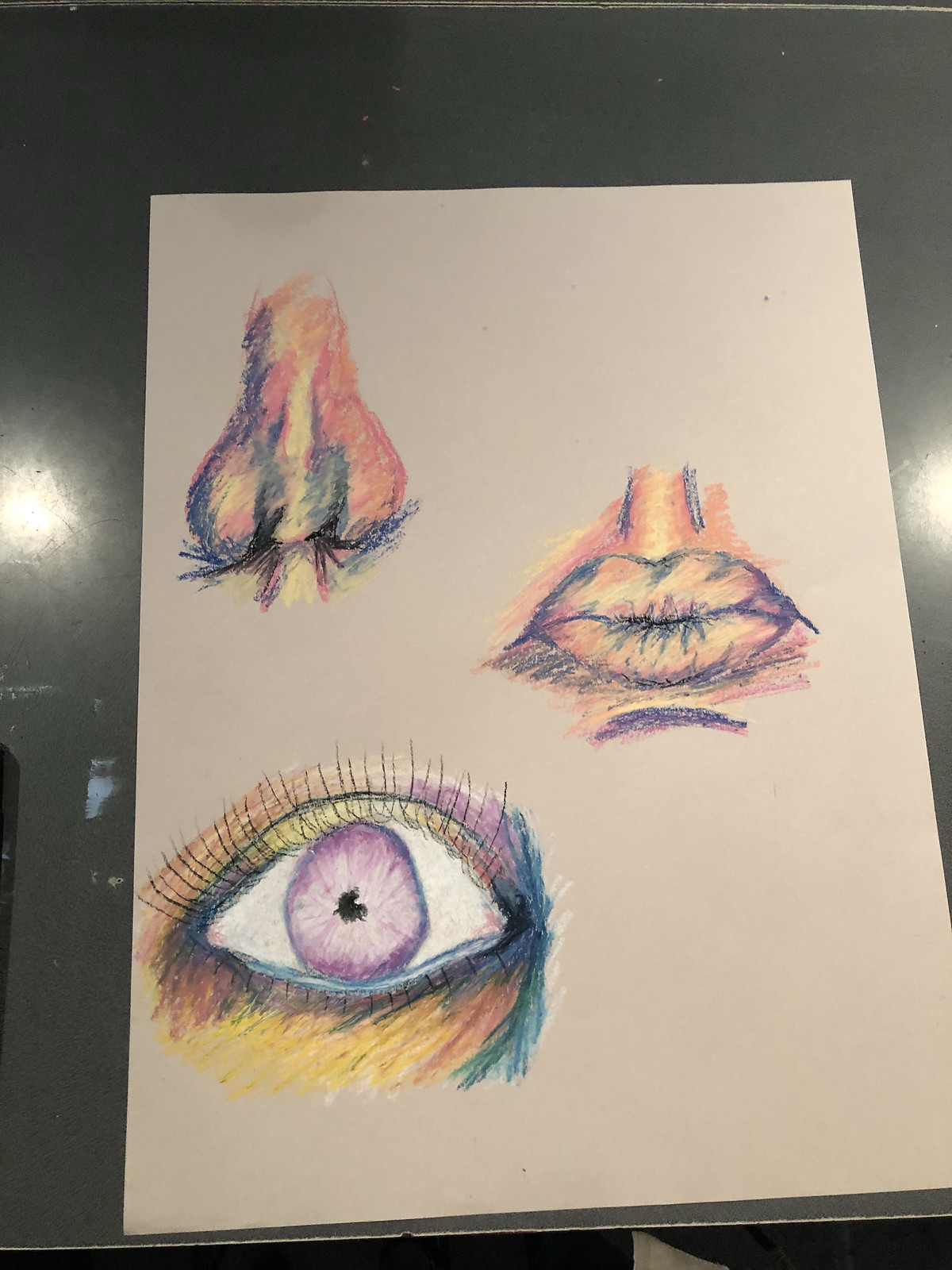The image showcases a hand-drawn artwork on what appears to be a slightly oversized piece of beige art paper or cardboard. The drawing, captured against a black surface, possibly a desk, includes three distinct and vividly colored facial features. At the top of the paper, there is a depiction of a nose, possibly paired with a mustache, crafted with meticulous detail. In the center-right of the composition, a pair of luscious lips is painted, exhibiting shades of light purple, teal, and yellow. The lower left corner of the artwork features a single eye, complete with lashes, irises, and pupils, rendered in harmonious hues of light purple, teal, and yellow. Each element - the nose, lips, and eye - is executed with vibrant colors, creating a striking contrast against the beige background of the drawing pad.